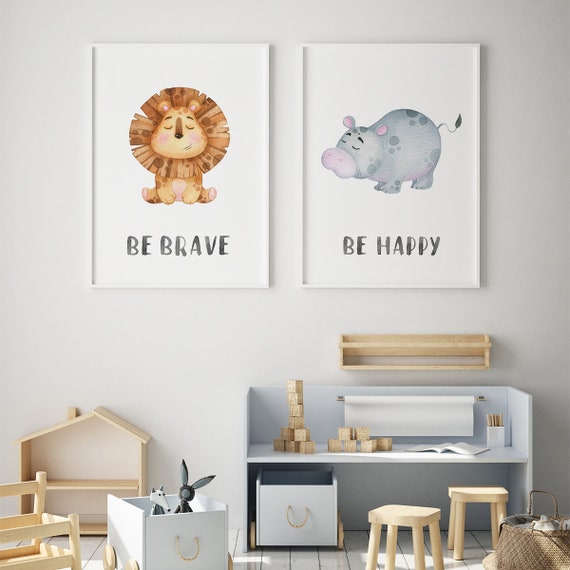This image depicts a cozy and charming nursery or children's room adorned with white walls. Prominently displayed on the wall are two large, white background screen prints. The left print features a cute baby lion with closed eyes and rosy cheeks, accompanied by the motivational phrase "be brave" in black letters. To the right, a cheerful baby hippopotamus with pink ears and a pink nose is depicted, with the words "be happy" inscribed below. Below these prints stands a simple wooden bookshelf or rail rack, empty of contents. A small desk sits in front of the rack, topped with wooden blocks, a white roll of paper, and flanked by two light-colored wooden stools. Additional details include a brown basket filled with assorted children’s toys, a wooden dollhouse affixed to the wall beside the desk, and a small bin on wheels situated underneath the desk.